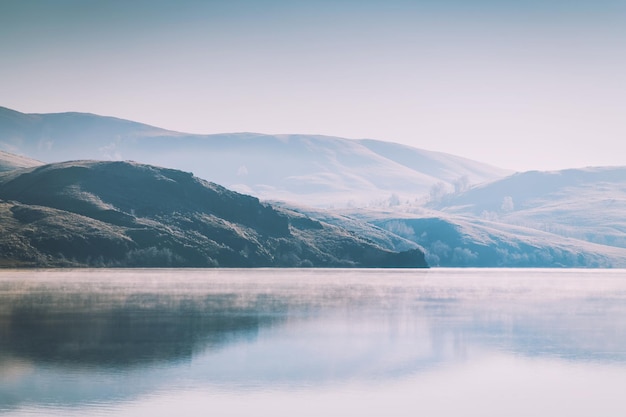The image depicts a serene outdoor scene captured during the daytime with a notable play of light and haze. Dominating the background are majestic, tall hills or mountains, which appear shrouded in a foggy haze, giving them a dreamlike quality. The sky above features patches of blue and areas of white, suggesting partial cloud cover. Below the hills, a body of water stretches across the foreground, reflecting the sunlight and appearing vibrant despite some darker, shimmering areas. The shoreline of the water is rough and textured, possibly hinting at rocky terrain. Trees and other plant life can be seen sparsely covering the hills, adding to the natural feel of the landscape. The overall atmosphere is tranquil and somewhat ethereal, enhanced by the hazy appearance which could suggest the image is a painting rather than a photograph.